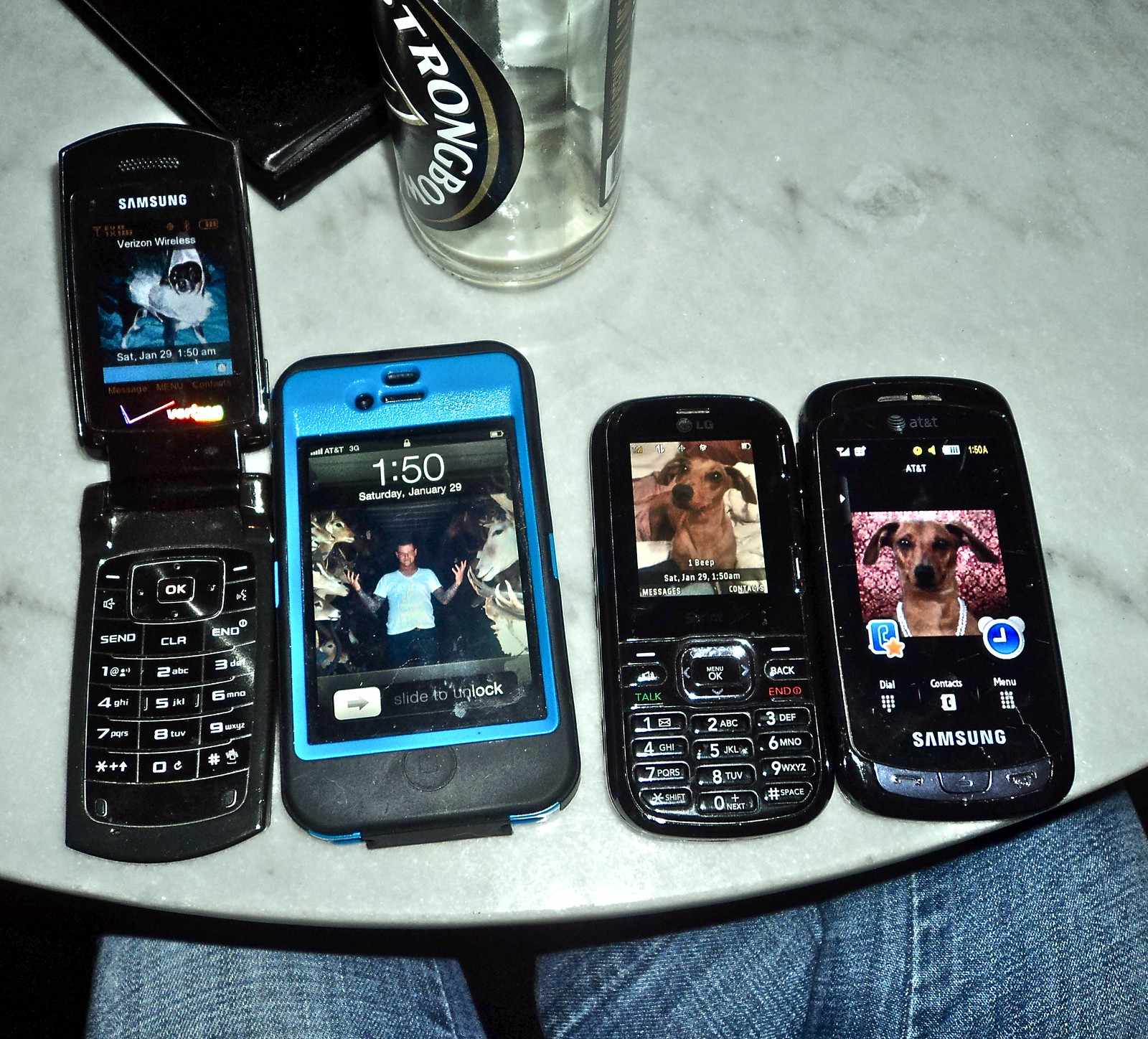The image showcases four different phones lined up in a row on a small table. At the bottom of the image, the photographer's jeans are visible. The table also has a black wallet and an empty bottle. Starting from the left, the first phone is a black Samsung flip phone branded with Verizon Wireless, displaying a wallpaper of a chihuahua in a costume with the date "Saturday, January 29th at 1:50 AM". The second phone is an early iPhone, likely a model 3 or 3G, encased in a blue and black cover. Its screen shows a quirky image of a person striking a pose among various animal heads, with the time "1:50" and the date "Saturday, June 29th" along with AT&T branding. The third phone is an older LG model, worn with age, showing a brown chihuahua or possibly a wiener dog on the screen with some of the text illegible due to wear. The fourth phone is another Samsung device, this time a very old AT&T touchscreen model, also featuring a background image of the same chihuahua against a pink and black background. The table, possibly a bed or coffee table, and the presence of the photographer's jeans suggest a casual, candid setting.